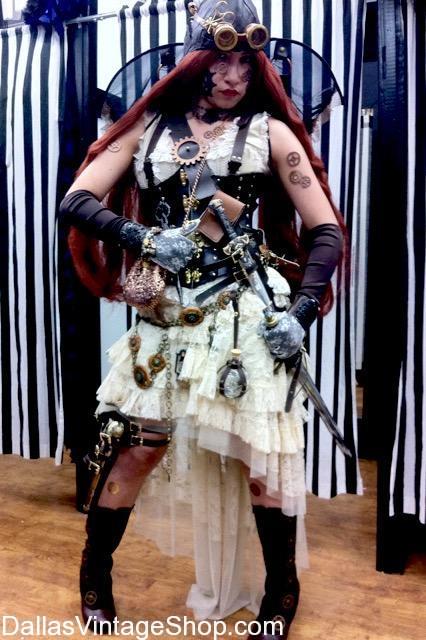This image features a woman in an elaborate steampunk cosplay, characterized by a blend of historical and fantastical elements. She is wearing a layered white lace dress evocative of vintage styles, overlaid with black leather and a black corset that cinches her waist. Her accessories include ornate chains, various gears, and a belt with a strap, enhancing the steampunk aesthetic. On her head, she sports a World War II-style leather pilot's cap and goggles, with her long, dark red hair cascading down her back.

The woman's left arm is adorned with several tattoos, featuring designs such as gears, and she has additional face paint that mimics intricate patterns like cobwebs or mechanical components. Black elbow-length gloves, decorated with French symbols, and sturdy black boots complete her ensemble. At her hip, she carries a detailed sword in a scabbard, and she is shown holding it with her left hand, ready to draw it at any moment.

The setting of the photograph is a dressing room with black and white cloth curtains on a rod, creating a contrasting background. At the bottom of the image, the text "DallasVintageShop.com" is prominently displayed, indicating the source of the costume pieces.